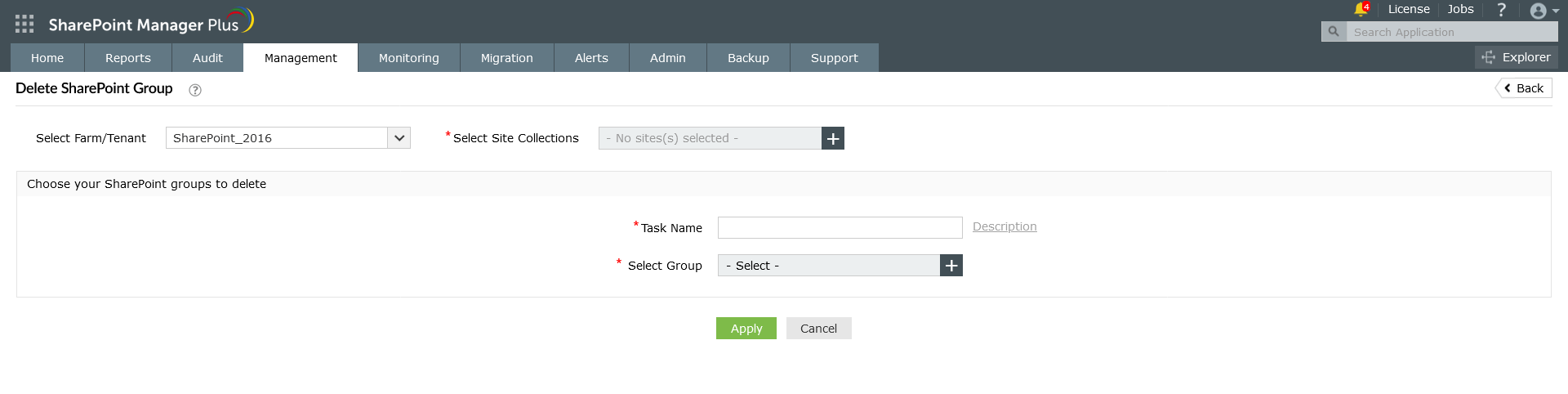This screenshot displays the interface of the SharePoint Manager Plus application. Prominently featured is a black rectangular box. In the top left corner of the interface, there is an array of nine small circles arranged into a 3x3 grid, creating a square shape. Adjacent to these circles, the text "SharePoint Manager Plus" is visible.

Beneath this text, a series of gray tabs stretch across the screen horizontally, labeled as follows: Home, Reports, Audit, Management, Monitoring, Migration, Alerts, Administration, Backup, and Support. The "Management" tab is currently selected, as indicated by its highlighted state. 

Within the Management section, the interface displays the heading "Delete SharePoint Group." Below this, a series of options appears. The first option, labeled "Select Farm/Tenant," is followed by a drop-down menu displaying "SharePoint 2016." 

Next, the section labeled "Select Site Connections" presents an empty input box, indicating that no connections are currently selected. Following this, the instruction "Choose Your SharePoint Groups to Delete" is shown. This is accompanied by two required fields, each marked with a red asterisk. The first is "Task Name," with an empty input box beside it. The second is "Select Group," featuring a drop-down menu currently labeled "Select."

At the bottom of the interface, two action buttons are displayed: "Apply" and "Cancel." No additional elements or content are present in the screenshot.